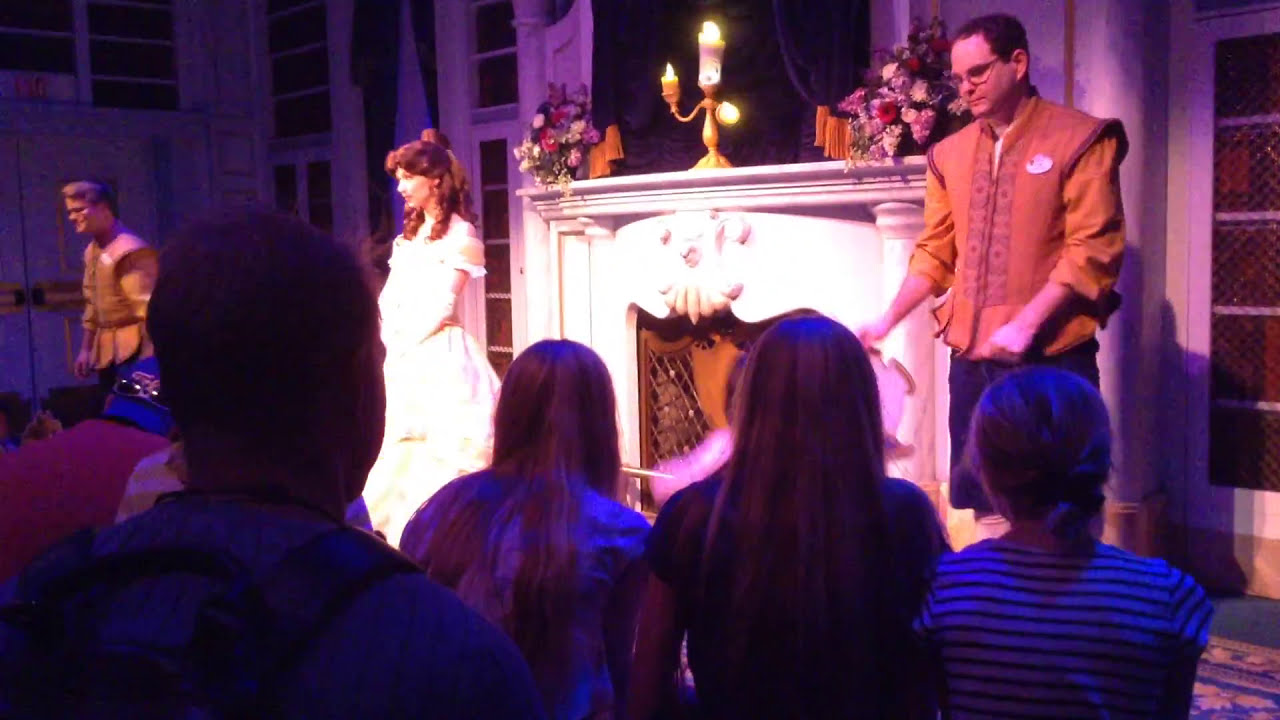In this detailed photograph of a stage play, the scene captures a live performance viewed from behind several audience members, who are engaged in the show. The ornate, white back wall with windows sets a grand backdrop for the stage, with an elegant white fireplace placed centrally. Atop the stage, a striking candlestick fitted with three LED lights takes the spotlight, framed by flowing curtains.

The performance features three actors: a woman in a white and yellow, off-the-shoulder dress stands prominently in the middle, suggesting she could be playing a character akin to Belle from "Beauty and the Beast." To her right is a man in a brown tunic paired with blue pants, possibly embodying a noble character. Another male actor stands to her left, dressed in an orange jacket shirt, contrasting against the backdrop.

Five audience members, possibly with more unseen, watch attentively, immersed in the unfolding drama. The combination of intricate stage design and vibrant costumes hints at a classical or fairy tale-inspired narrative.